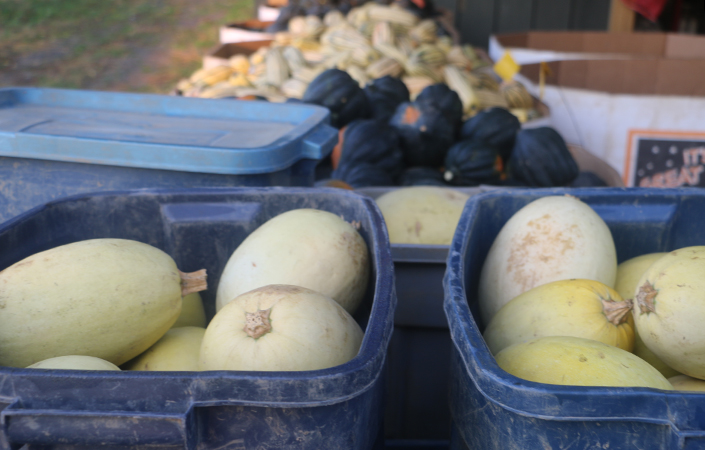The photograph depicts a vibrant scene at a fruit market. In the foreground, two large dark blue plastic tubs sit open, brimming with pale yellow, oval-shaped gourds, each adorned with tiny, light brown stems. One of the tub lids is visible to the left, providing a contrast to the orderly chaos of the gourds within. Slightly further back, out of full view, there is another tub filled with similar gourds, and behind this, a closed blue container can be seen.

The background reveals an assortment of other fruits and vegetables, including dark blue colored fruits, yellow bananas or squash, and various types of squash in different hues and shapes. Completing the rustic scene, a large white cardboard box sits to the right, adorned with a sign featuring an orange border and white stars, stating part of a phrase: "it's great," in bold orange lettering against a black background. To the left, a grassy path hints at the outdoor setting, enhancing the market atmosphere.